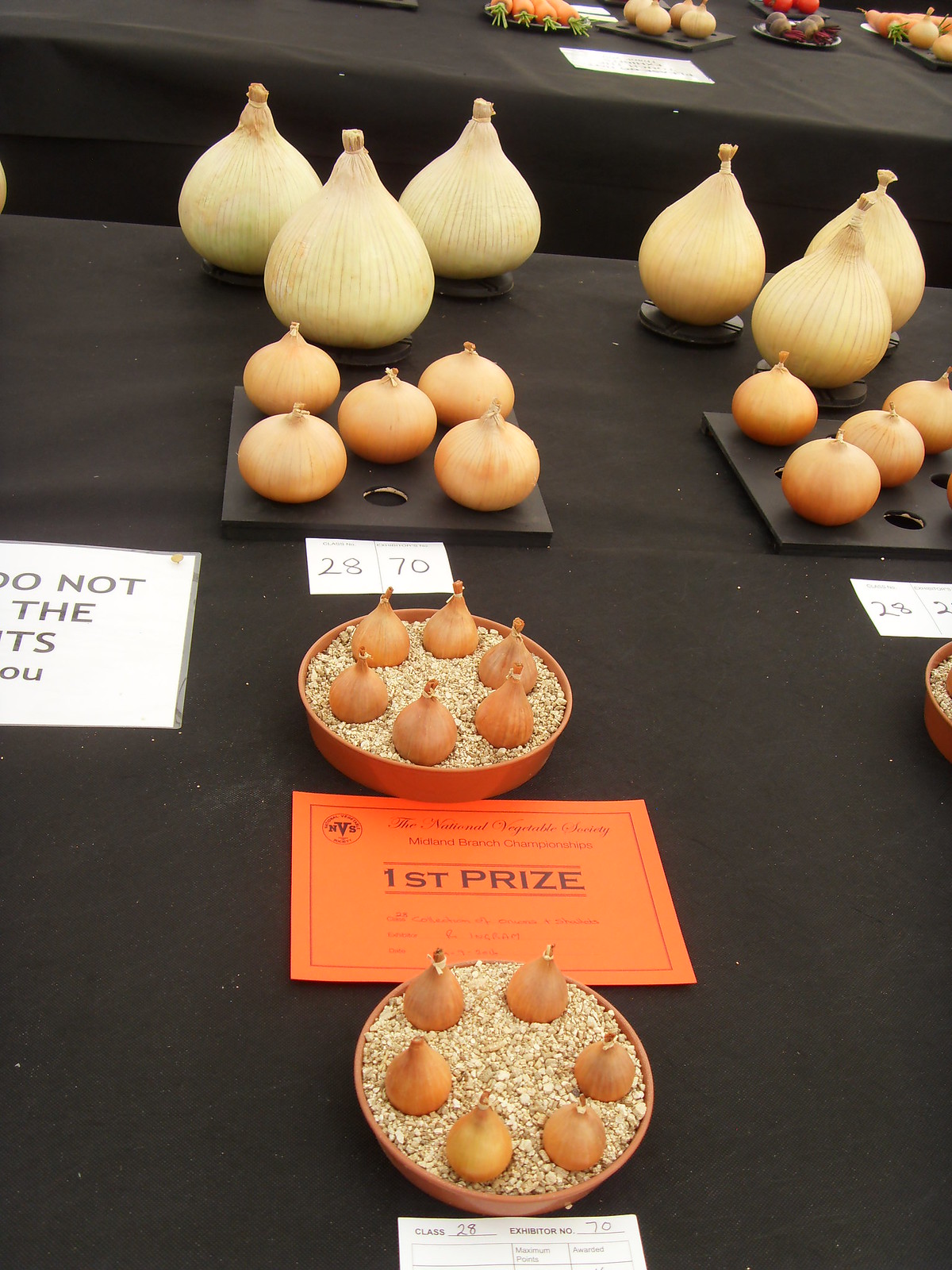The image depicts a black tablecloth background at what appears to be a state fair or a similar competition. Centered from top to bottom are meticulously arranged vegetables, predominantly onions and garlic. At the very top, three large yellow onions stand out, positioned on their round sides with their tops pointing upwards. Beneath them, five somewhat smaller, orange-colored onions are neatly lined up. Below these is a piece of paper displaying the numbers "28" and "70".

Continuing downward, there is an orange bowl filled with smaller orange onions resting on what resembles a bed of rice. Below this bowl, an orange card bearing the inscription "first prize" in black ink is prominently displayed, indicating a competition setting. Flanking this arrangement, to the left and right, are white pieces of paper with black lettering. The paper on the left has partial text saying "do not the something," while the one on the right contains numbers alongside more vegetables. The entire scene is echoed nearby with similar bowls and arrangements, suggesting a repeated pattern of onion displays, all contributing to the sense of a well-organized vegetable competition.